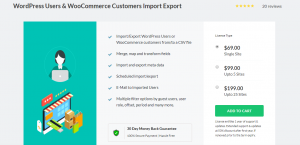The image is a small, blurry screenshot of a web page. On the left side, there is a green box featuring an image of a woman working on a computer. Below this, there appears to be an illustration of a storefront window alongside clip art images of credit cards, boxes, and shopping bags, seemingly placed at random.

The text within the image is difficult to read, but key phrases that can be discerned include "WordPress users," "commerce," and "WooCommerce customers import export." 

On the right-hand side of the page, there are options for selecting a license type. The choices visible are priced at $69, $99, and $199, with the $69 option currently selected. Beneath these options is a green button labeled "Add to Cart."

The center of the page seems to contain a list of features offered by a product or service, and there's an indication of a "30-day money-back guarantee" towards the very bottom. Overall, the details are quite blurry, making it challenging to read the finer elements.